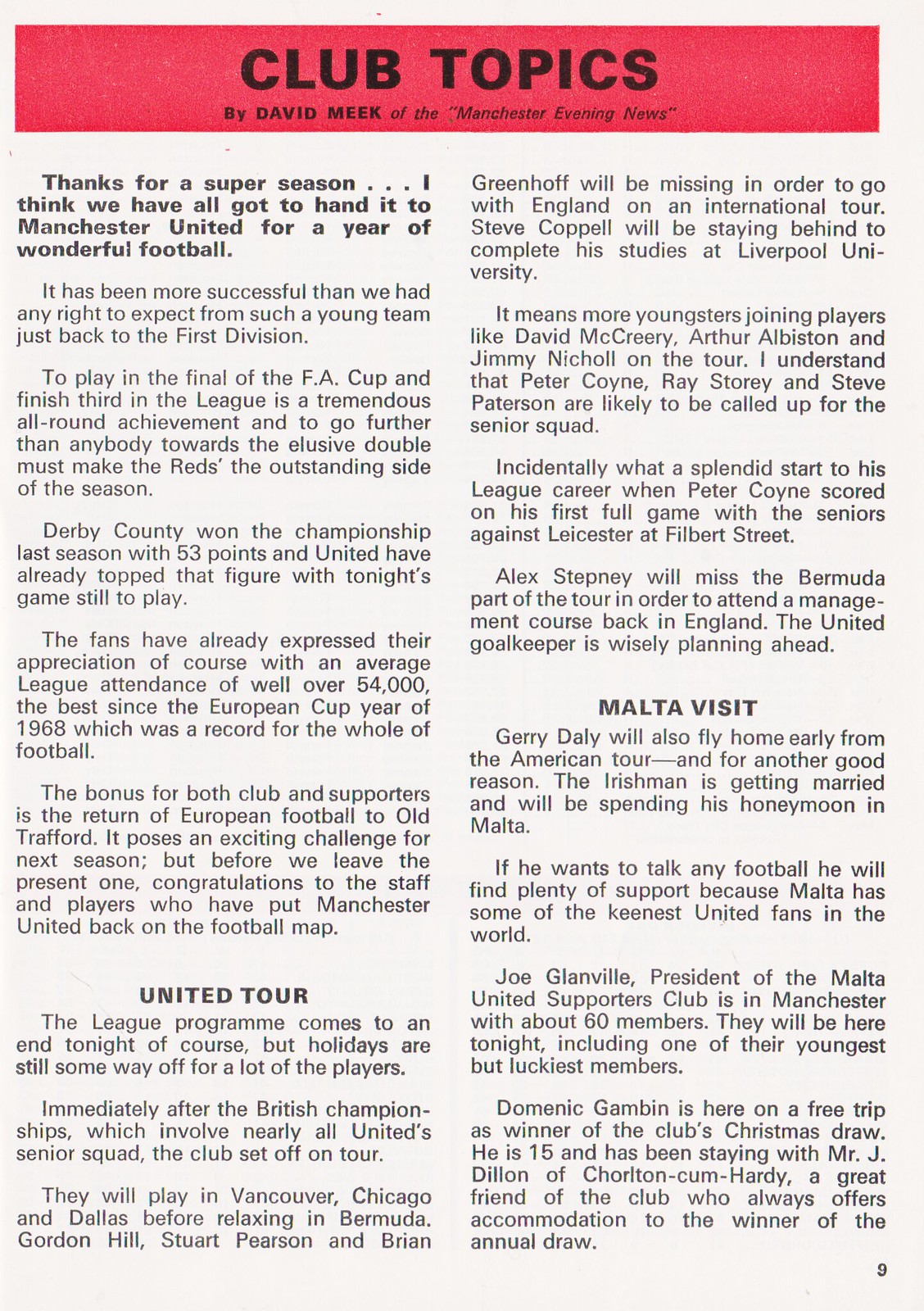This image is a black-and-white photograph of a newspaper article from a magazine or book, featuring a light red border at the top with "Club Topics" in black font, authored by David Meek of the Manchester Evening News. The two-column article starts with the bolded text "Thanks for a super season," commending Manchester United for their remarkable football year. Despite being a young team recently promoted to the first division, they played in the FA Cup final, finished third in the league, and exceeded last season's championship points. Their success attracted average league attendances of over 54,000—the highest since 1968—and secured a return to European football at Old Trafford. Another section, under the subheading "United Tour," discusses the club's post-season tour to Vancouver, Chicago, and Dallas, with notable absences for international duty and studies, highlighting players like Peter Coyne and Alex Stepney. The final subheading, "Malta Visit," details Gerry Daly's upcoming marriage and honeymoon in Malta and the enthusiastic support from the local United fans, exemplified by 15-year-old Dominic Gambon, a club Christmas draw winner visiting Manchester.